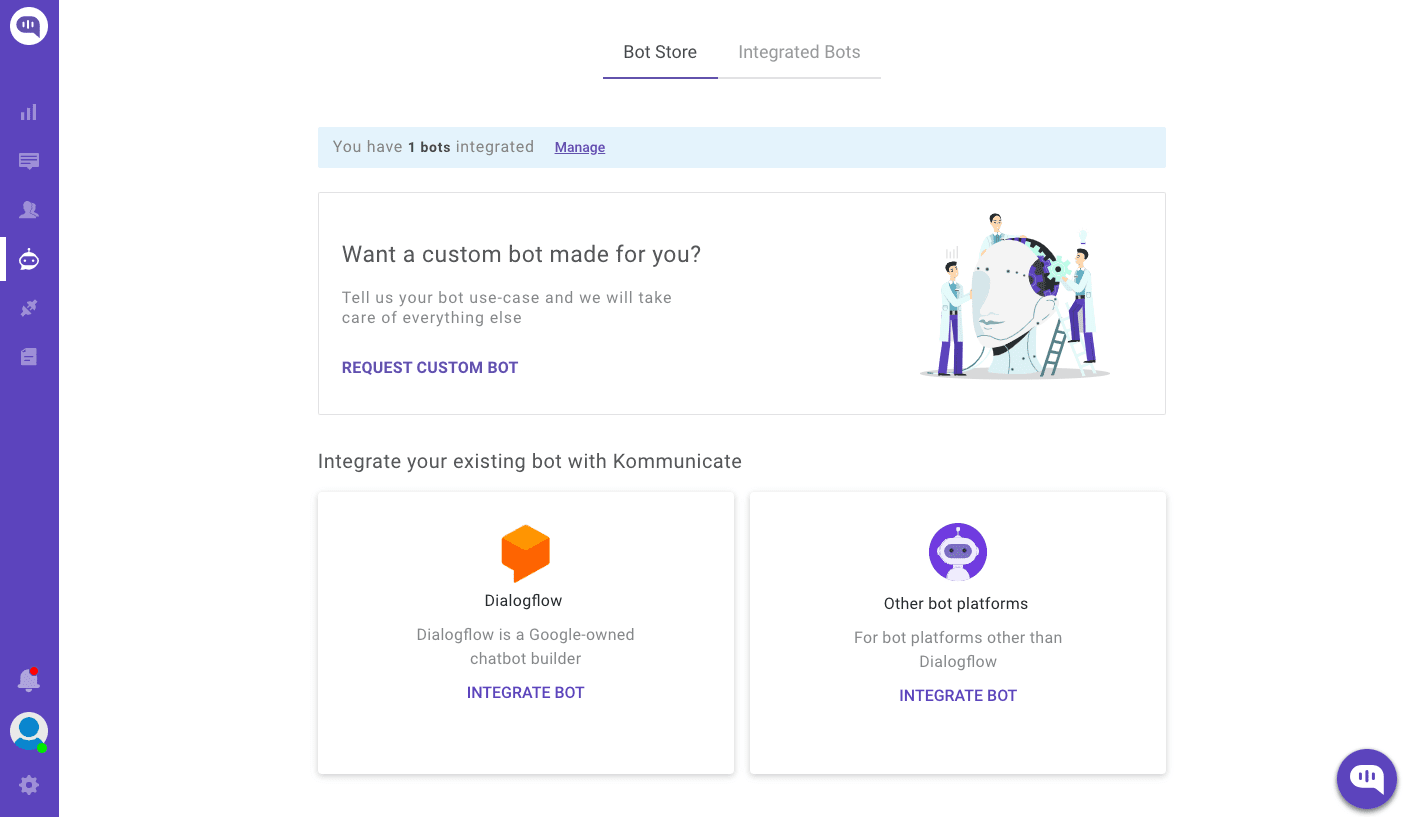The interface features a sleek, purple-striped navigation bar on the left side of the screen. At the top of this bar is a white circular icon resembling a conversation bubble, filled in with purple. Below it, three bars arranged from smaller to larger represent different menu sections. The icons proceeding downward include a text bubble, a contacts symbol, one that looks like the Reddit logo, a plugin icon, and a document symbol. At the bottom, there is a notification indicator with a red dot, a profile icon with a blue person and a green dot, and a settings gear.

In the central part of the interface, bold text reads "Bot Store" and "Integrated Bots." "Bot Store" is underlined in blue. A message below mentions, "You have one bot integrated," with the word "manage" highlighted in blue and also underlined. This text appears on a light blue background strip.

Below this, a large horizontal rectangle contains the text: "Want a custom bot made for you? Tell us your bot use-case and we will take care of everything else." A call to action, "Request custom bot," is highlighted in blue. To the right of this text, an illustration depicts three individuals working on the head of a robot. Underneath this image is the text, "Integrate your existing bot with Communicate," carefully spelled out for clarity.